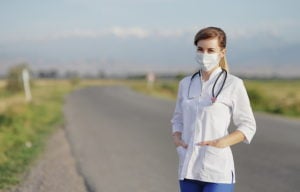In this slightly blurry image taken on a very sunny day, a Caucasian woman stands on a rural road. She appears to be a doctor, nurse, or medical worker, evidenced by her white quarter-length sleeved shirt buttoned up to the top, blue trousers, stethoscope around her neck, and white surgical mask covering her face. Her brown hair is pulled back into a ponytail. Positioned slightly toward the right side of the image, she is captured amidst a picturesque rural backdrop. The winding road in front of her stretches from the bottom of the picture toward the middle, curving sharply to the right. Surrounding this road are open fields with patches of grass, tree lines at a distance, and what looks like farmland extending into the horizon. Towards the far distance, small trees are visible, and a majestic mountain range with snow-capped peaks can be seen under a clear blue sky adorned with a few white clouds. The overall scene, filled with colors of yellow, green, sky blue, gray, brown, light blue, white, black, and beige, paints a serene and detailed countryside setting.